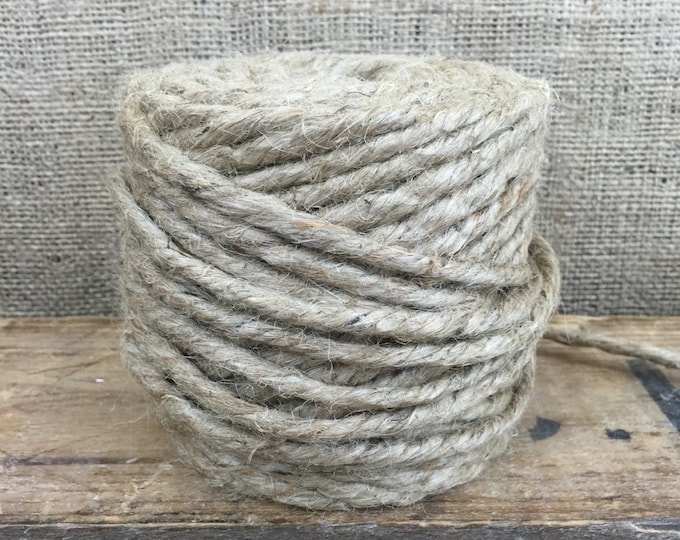The image features a close-up view of a ball of heavy twine, centrally positioned on an aged, brown wooden ledge, possibly a table or shelf. The twine, which has a straight-sided, uniform shape with a very straight top, is an oatmeal or light beige color, suggestive of a natural material such as jute, sisal, or rope. No text appears in the image. The twine takes up the majority of the picture. In the background, there is a white mesh or natural light-colored burlap material that contrasts with the dark, rustic wood below. The setting has a DIY aesthetic. The texture and positioning suggest that the twine is new, with the end of the rope extending out of the frame.